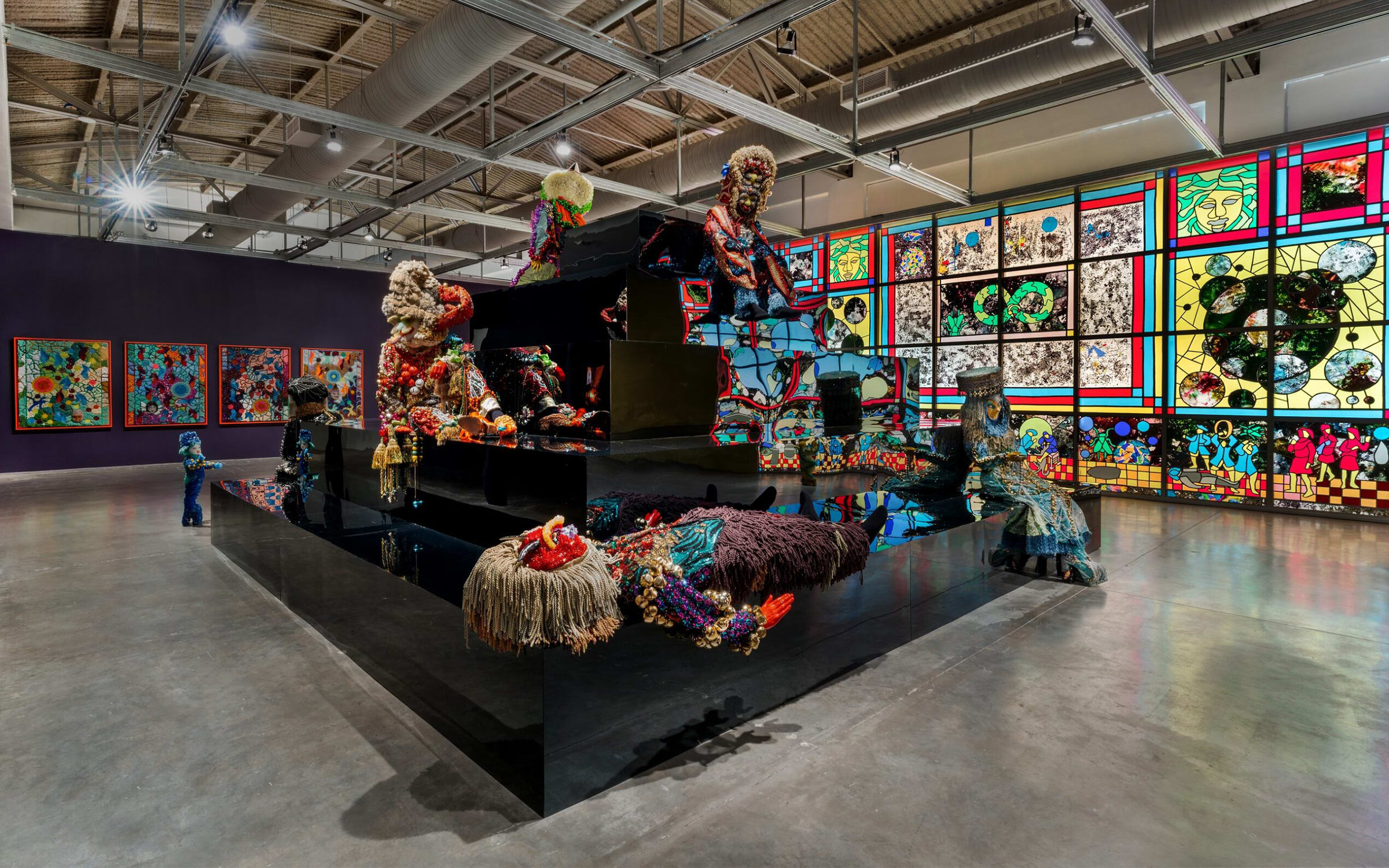This rectangular landscape photograph captures a vibrant art gallery interior. At the center stands a striking black structure adorned with various art sculptures, seemingly human-like in form and crafted from what appears to be papier-mâché. These sculptures are rich in color, featuring hues of purple, blue, yellow, orange, and red, adding an eclectic burst of vibrancy to the scene. On the left side of the image, a dark gray wall serves as the backdrop for four abstract paintings, each evoking floral motifs in a distinctive and imaginative style. On the right side, a large stained glass window, intricately designed with diverse patterns, allows colorful light to filter through, enhancing the artistic ambiance of the gallery.